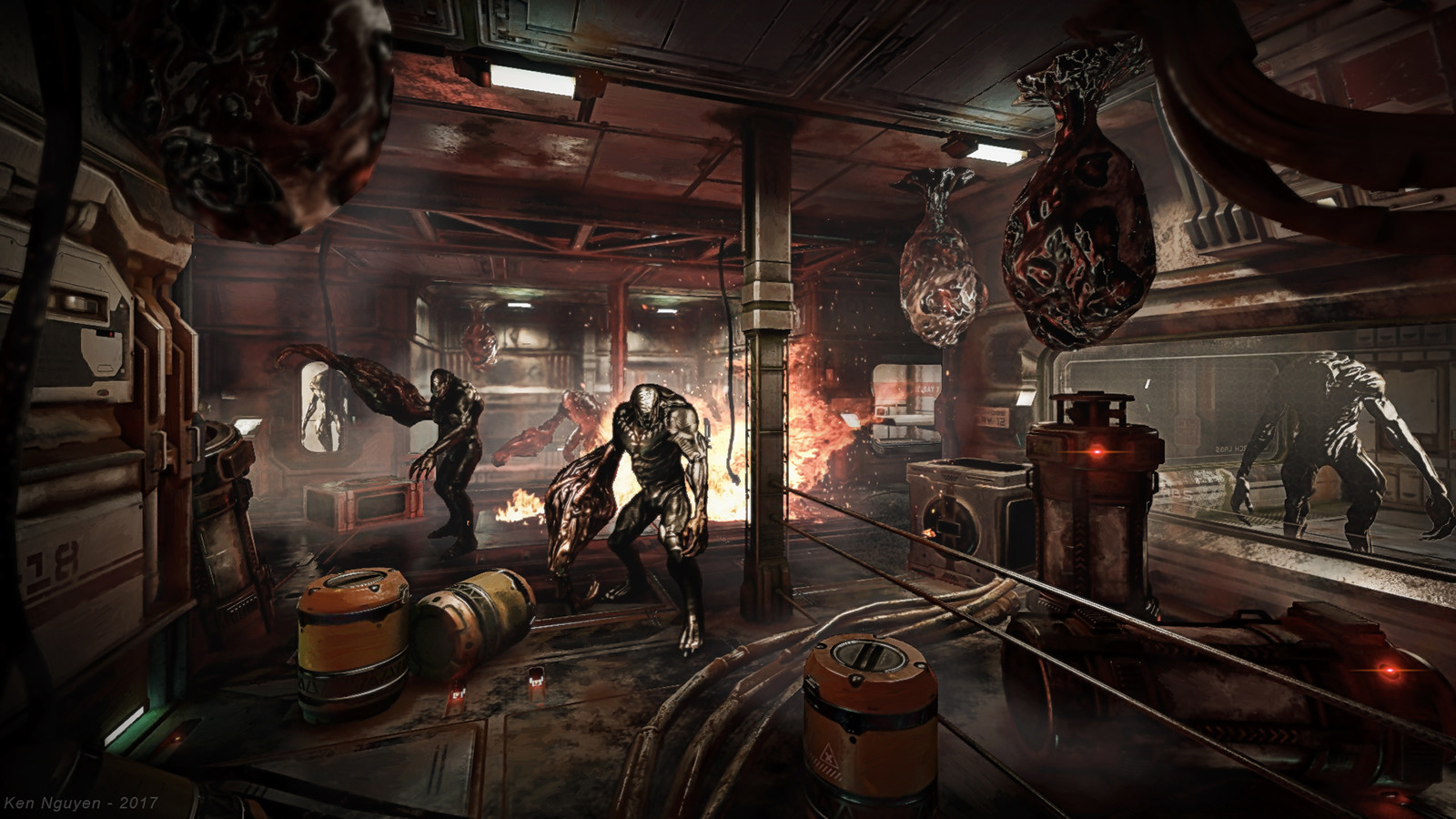The image depicts an atmospheric scene that seems to be a still from a video game, likely designed within the past 15 years, showcasing a dark, metallic spaceship interior. The environment is characterized by its metal-clad floors, ceilings, and walls, which are detailed with drawers, handles, and futuristic borders, evoking a high-tech, industrial feel. Central to the scene is a muscular, gray-skinned, alien creature with an exceptionally large and possibly weaponized right arm. This creature is situated amid a clutter of cylindrical metal barrels and smaller orange battery-like containers strewn across the floor.

Multiple similar alien entities are present, one directly facing the camera while others are scattered around—one reaching towards the wall and another visible through a rectangular glass window on the right side of the room, which serves as an observation area. Suspended from the ceiling are large, fleshy, cocoon-like structures, hinting that these monsters might emerge from them. The cocoons are shiny and textured, giving off a gory, organic vibe.

In the midst of the room, a fire burns brightly, casting an eerie glow and creating an atmosphere filled with smoke and sparks, further accentuating the chaotic and dirty appearance of the setting. The scene might be at a crossroads within the spaceship, intensifying the sense of suspense and action typical of a high-paced video game environment.